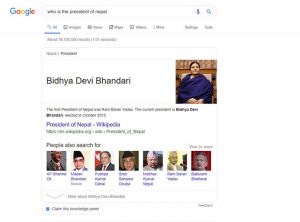This image shows a Google search results page generated by the query "What is the president of Nepal?" At the top, there is a prominently displayed information box featuring a photograph of the current president, Bidhya Devi Bhandari, along with concise details about her. Directly below this box is a link to her Wikipedia page, listed as one of the top results. 

Further down, there is a section titled "People also searched for," displaying a row of seven photographs of various male leaders from the region. The text beneath these images is slightly blurry, making it difficult to read even when zoomed in. On the left side of the information box is a speech bubble containing some additional text.

The Google logo is visibly placed on the far left of the search bar, while on the far right end of the search bar, there is a microphone icon and a search icon.